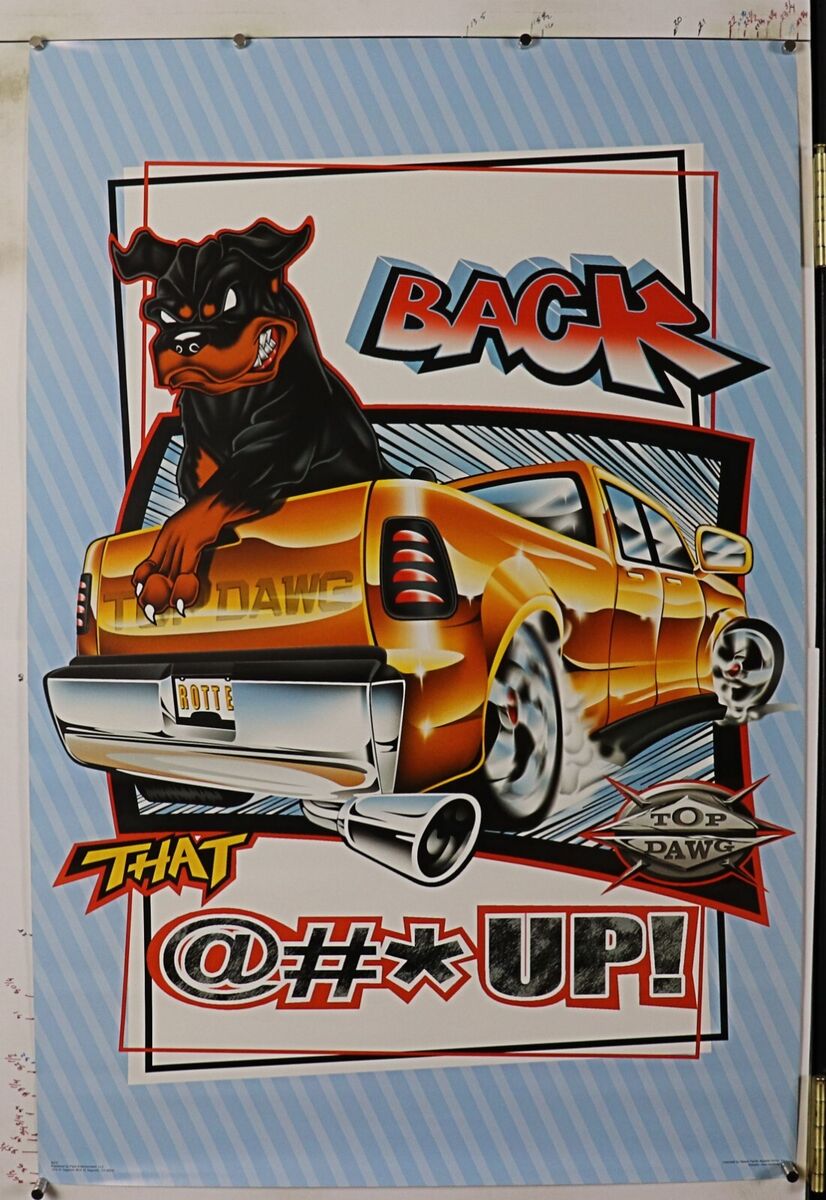This is an image of a rectangular poster with a clean, detailed graphical illustration, pinned onto a white wall using multiple nails—four at the top and two at the bottom. The poster features a striped, diagonal pattern in light blue and white shades, creating a vibrant background. Central to the poster is a shiny, new, orange pickup truck with a metallic, silver-glossy finish on the windows and a black-lined outline, evoking a cartoony appearance. Inside the truck's bed sits a large, animated Rottweiler, depicted in black and brown, gritting its teeth menacingly. The truck's license plate reads "ROT," emphasizing the dog's breed, while text above the truck in graffiti-style black, red, and white font says, "BACK THAT @#$% UP!" Below the truck, in a graffiti style as well, is the phrase "TOP DOG," reinforcing the dominant theme of the artwork. The scene is accentuated by a sense of motion, suggested by wisps of smoke around the truck's tires, imparting a dynamic feel to the image.